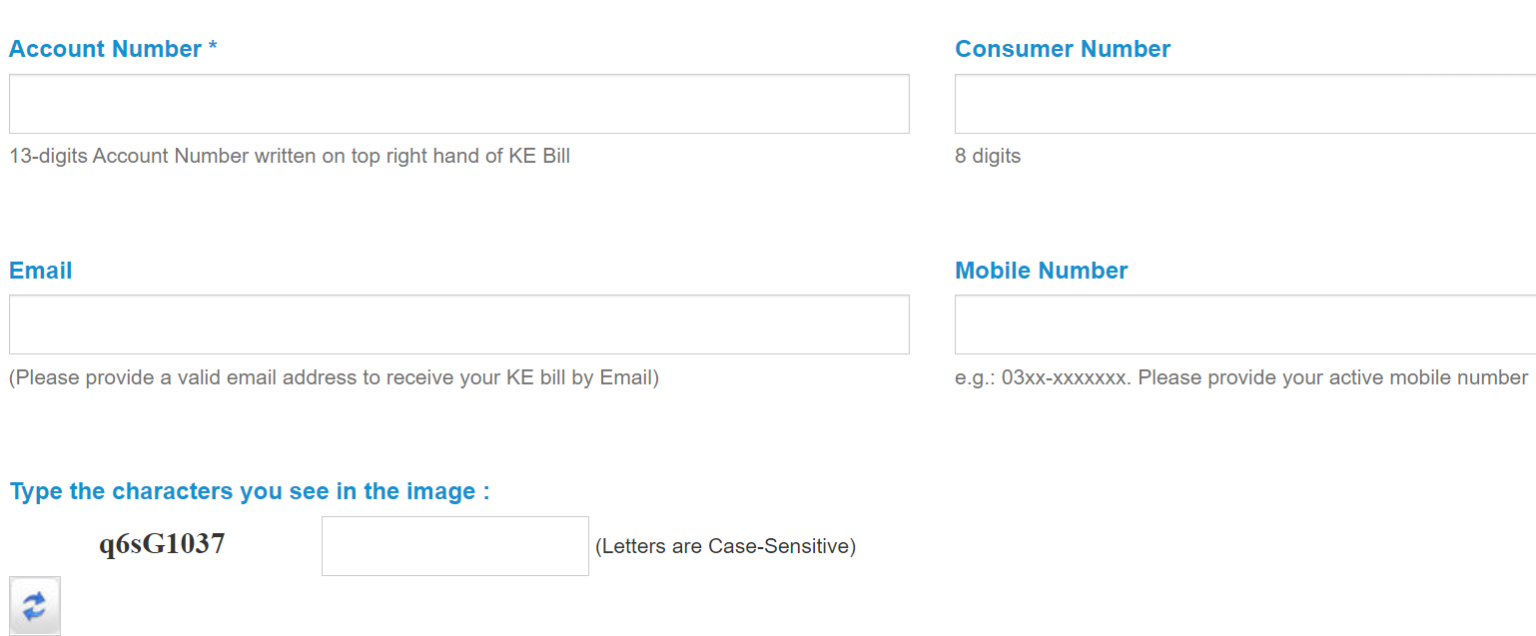This image is a screenshot of the personal information section of a website, displayed on a white background in a structured format from left to right, top to bottom. 

At the top in blue text, it reads "Account Number" followed by a blue asterisk. Beneath this, there is an input box to enter the account number. Under the box, the text "13 digits account number written on the top right hand of K E bill" is displayed in gray.

To the right, "Consumer Number" is written in blue text with an associated input box directly below. Under this box, it states "8 digits" in gray text.

Below these fields, on the left side, it reads "Email" in blue text with an input box underneath for entering an email address. An informational note follows in parentheses: "Please provide a valid email address to receive your K E bill by email."

On the right, "Mobile Number" is written in blue text with an input box below. Beneath this box, instructions are given in gray: "E.g. 03XX-XXXXXXX Please provide your active mobile number."

Further down, "Type the characters you see in the image" is displayed in blue, with a distinct captcha code - ‘q6sG1037’ - highlighted in bold. To the right of this captcha image is an input box for entering the characters, alongside the note "letters are case sensitive."

Finally, at the bottom left of the screenshot, there is a gray box containing arrows pointing to the right and left, likely for navigation purposes.